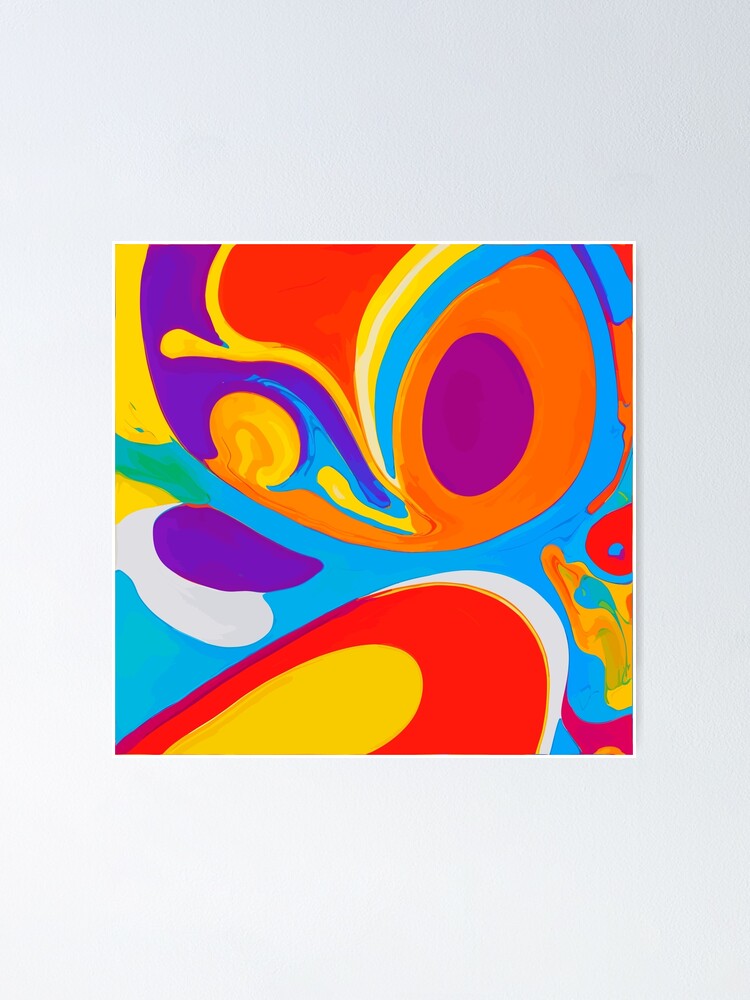Here we have a vibrant, abstract painting set within a portrait-oriented light gray or white background, creating a striking contrast. The central image is a square filled with swirling, organic shapes and vivid colors, predominantly featuring reds, yellows, purples, oranges, blues, and whites. At the bottom, a yellow oval capped with a red U-shape and white crescent stands out. Blue swirls through the middle, adding movement, while a prominent circle with a purple center encircled by orange and outlined by blue and yellow emerges at the top right. The painting, which could be perceived as digital or handmade, is lively and open to interpretation, possibly even suggesting a face with eyes, a nose, and fingers in its vibrant, flowing patterns.